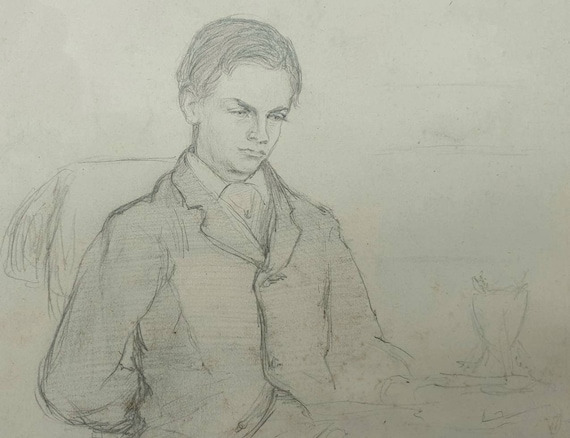This detailed pencil sketch, likely created on a faded piece of vellum or bristol paper, depicts a young man from an earlier era. He sits in a chair, perhaps at a desk, dressed in a buttoned-up suit jacket with a high-collared white dress shirt underneath. His short, wavy brown hair complements his forlorn expression as he looks downward, immersed in deep thought or contemplation. His left hand is resting on a table beside a vaguely sketched glass or stand, while his right arm appears to be behind his back or in his pocket. The background hints at a chair's pillow or backing, adding to the melancholic atmosphere of the scene. The sketch artist employs subtle shading and lines to convey the somber mood, with the old-fashioned attire suggesting a historic setting. The boy's light eyes and brooding demeanor provide a poignant focal point, inviting viewers to ponder the story behind his subdued expression.